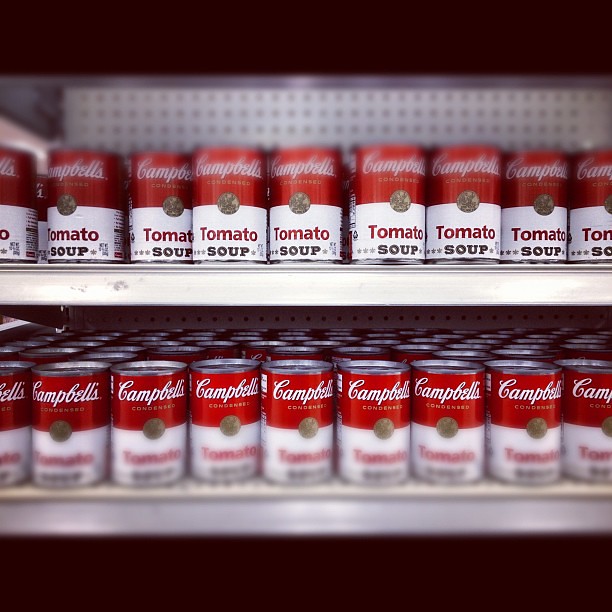The image depicts a section of a grocery store's soup aisle, showcasing two white metal shelves against a perforated white backboard. Both shelves are neatly stocked with rows of Campbell's condensed tomato soup cans, each row containing about 10 cans, aligned perfectly and facing forward. The cans have a distinctive design: the top half is red with the cursive Campbell's logo in white, accompanied by the word "condensed" beneath it. A gold seal decorates the center, overlapping the red and white border. Below the seal, in the white bottom half of the can, the words "tomato soup" are prominently displayed, with "tomato" in red and "soup" in bold black letters. Three small stars flank the word "soup" on each can. The bottom halves of the cans on the top shelf and the top halves of the cans on the bottom shelf are particularly clear and in focus, adding to the uniformity and precise organization of the display.